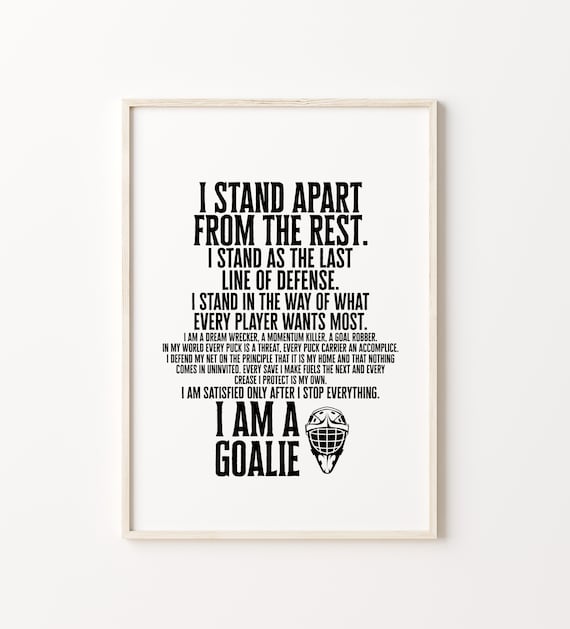The image depicts a framed picture mounted on a white wall. The off-white wooden frame, made from timber, is light brown and casts a shadow to the right. Inside the frame, a white poster contains a powerful text written in black letters starting out large and gradually becoming smaller, with "I am a goalie" emphasized at the end in the largest text. The text reads: "I stand apart from the rest. I stand as the last line of defense. I stand in the way of what every player wants most. I am a dream wrecker, a momentum killer, a goal robber. In my world, every puck is a threat. Every puck carrier an accomplice. I defend my net on the principle that it is my home and that nothing comes in uninvited. Every save I make fuels the next in every crease I protect with my own. I am satisfied only after I stop everything. I am a goalie." Adjacent to this text is a simple silhouette clipart of a hockey mask, reinforcing the goalie's narrative.